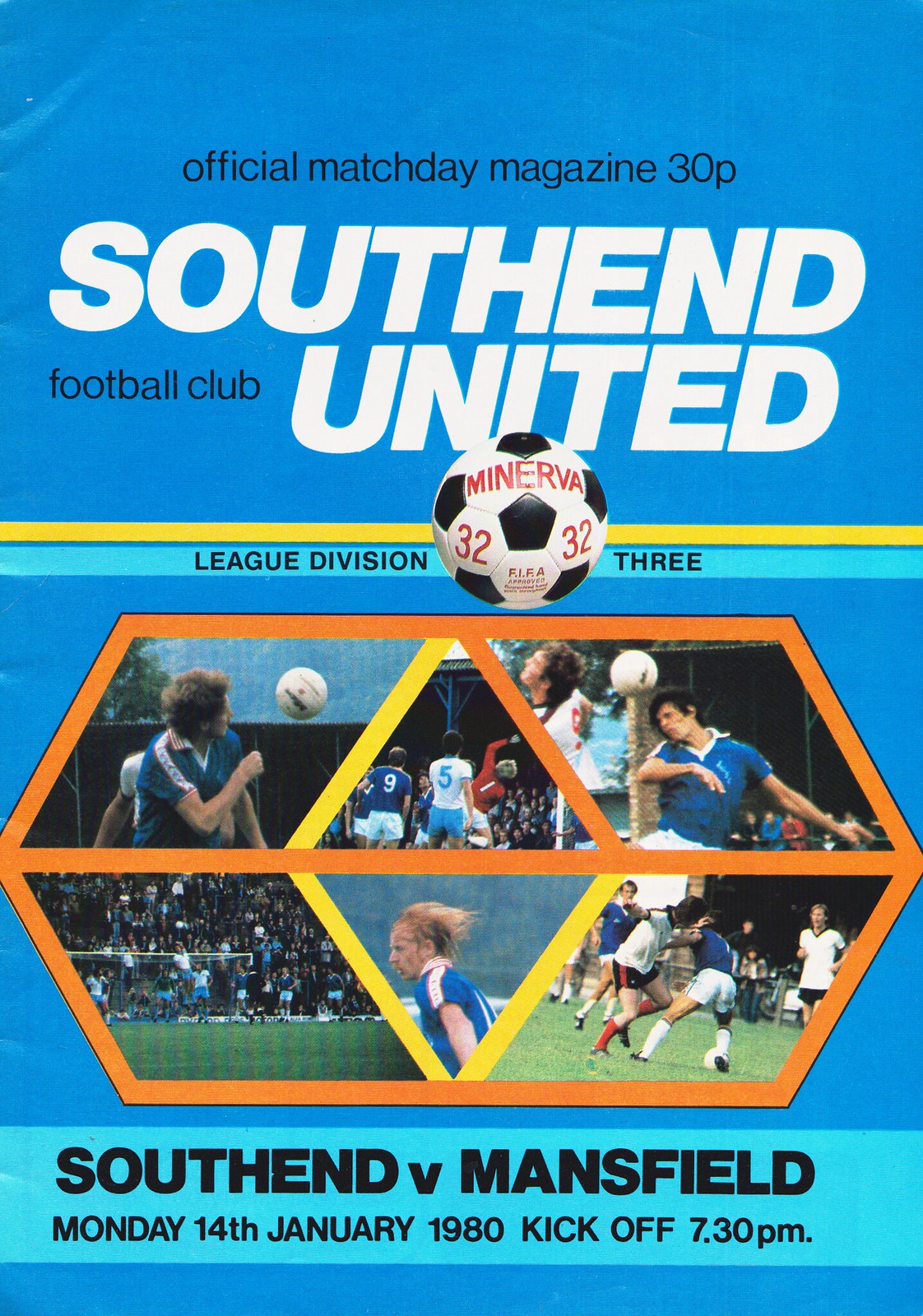The image is the front cover of a soccer match program with a vibrant blue background. At the top, in small, all-lowercase black font, it reads "official match day magazine 30p." Below this, in large, bold white capital letters, it says "SOUTH END UNITED," with "football club" in smaller black lowercase letters to the left. A classic black-and-white soccer ball adorned with red lettering "Minerva 32" sits prominently in the center, intersected by a horizontal yellow stripe. Below the ball, there's a light turquoise stripe with the inscription "League Division III." The middle third of the cover features an intricate design of a soccer ball made up of multiple prisms, each containing a photo of players in action. At the bottom, a turquoise banner details the match information: "South End vs. Mansfield, Monday, 14 January 1980, kickoff at 7.30pm."